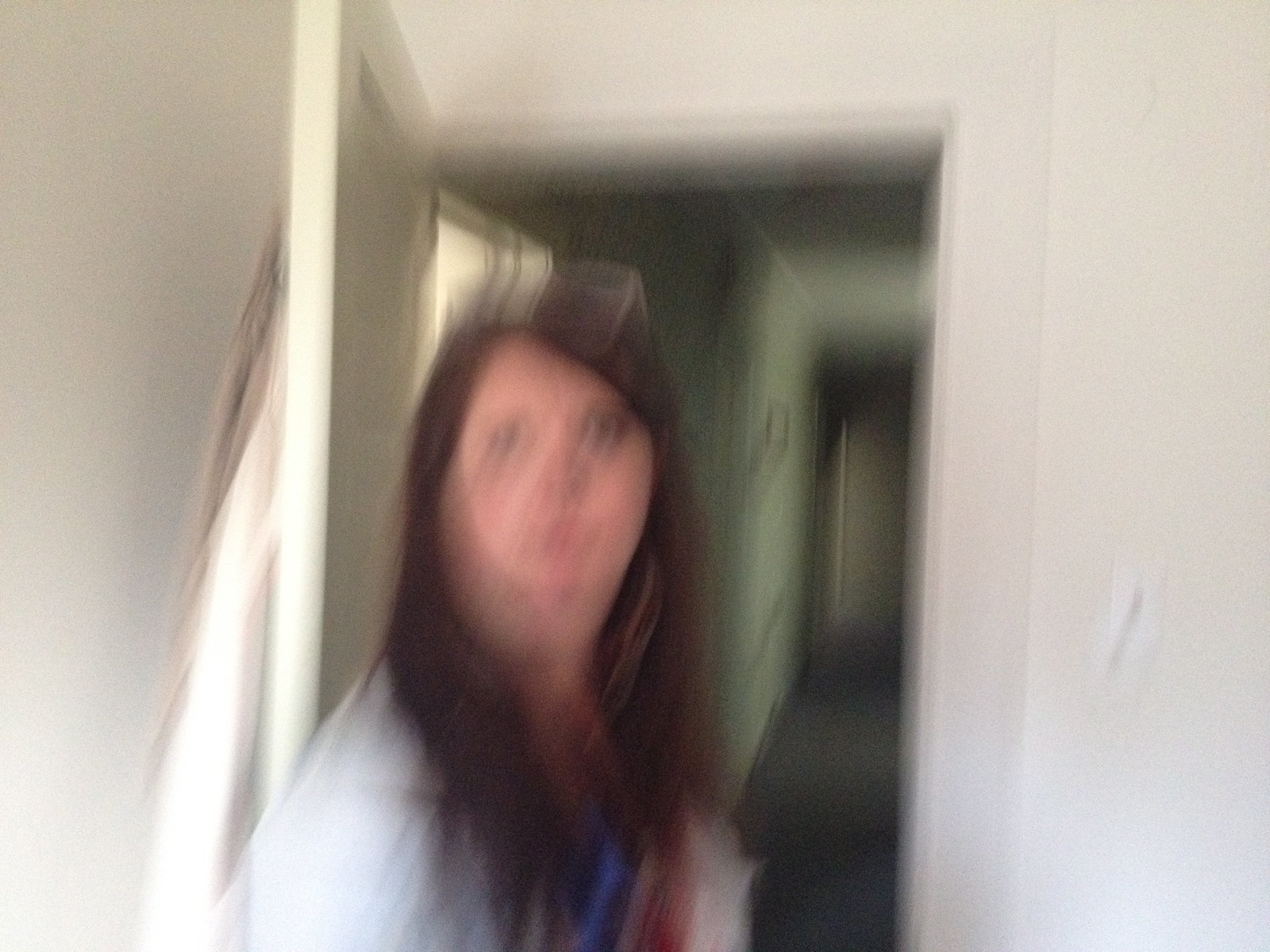The photograph is extremely blurry, capturing a close-up of a woman standing in an open doorway. The woman's long brown hair cascades past her shoulders, framing her indistinct facial features, although she appears to have brown eyes and a pair of glasses resting on top of her head. She is wearing a white blouse, with what seems to be a blue shirt underneath, and possibly a touch of red lining her attire.

The setting is dominated by an out-of-focus background, which appears to be a light green hallway with a narrow gray walkway. At the far end of the hallway, a gray door is visible, possibly adorned with a mirror. Directly behind the woman, the open door she stands next to has fabric items hanging on it, including a white article. Above her head, a window is faintly visible, flanked by white and green curtains. The overall image, despite its lack of clarity, hints at a domestic interior with scattered details contributing to its depth.